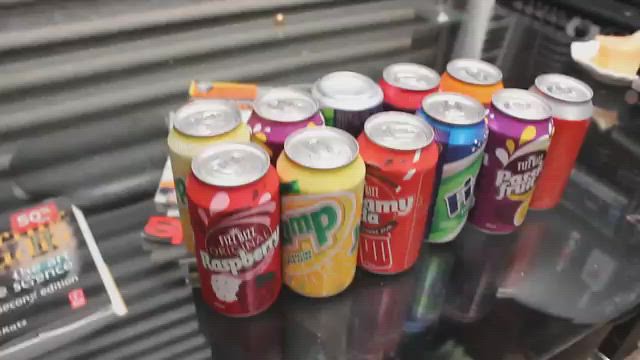The blurry, wide-angle photograph captures an assortment of unopened 12-ounce soda pop cans arranged on a glass shelf, which appears to be situated in an environment resembling an office break room. In the foreground, six cans are positioned in a row sloping away from left to right at an angle of about 20-30 degrees. The first can displays "Fizz Bizz Original Raspberry" with red and pink colors, followed by a yellow and green can with an unreadable label. Next to it is a red and brown can, then a multi-colored blue, white, green, and black can, whose label is also unreadable. The fifth can is purple, white, and yellow, labeled "Fizz Bizz Passion Fruit," and the last can in the front row is silver and red, lacking a visible label. A second row of soda cans is partially obscured by the first, with visible colors including yellow, purple, black and green, red, and orange. Notably, the third can from the left is upside down. None of the cans have been opened, and they all have silver pop-tops. To the left of the cans, there is a textbook titled "The Art of Science: Second Edition." In the top right corner of the image, a white dish is faintly visible, and the background consists of out-of-focus gray shelves and horizontal bars.